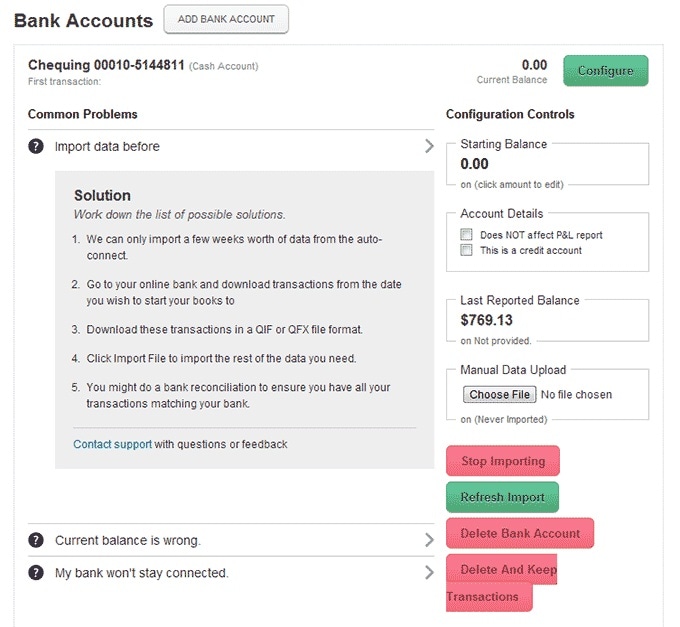The image displays a user interface of a banking application. In the top left corner, there is a section titled "Bank Accounts," and to the right of this title is an "Add Bank Account" button. The background is predominantly white, with a light gray box centered in the middle of the photo. Scattered throughout the image are various buttons in colors such as green, red, and gray. 

A specific checking account is visible, and interestingly, it uses the British spelling "cheque" which suggests that this might be an international or non-US account. Below the account information, there are several options and buttons for users to address common problems, configure controls, and select help topics. Available help options include issues like "The current balance is wrong," "My bank won't stay connected," among others.

Further down, we can see details like the current balance, the starting balance, the last reported balance, and options for manual data upload. Additional functions include "Stop Importing," "Refresh Import," "Delete Bank Account," "Delete and Keep Transactions," and "Configure." The account is identified as a cash account.